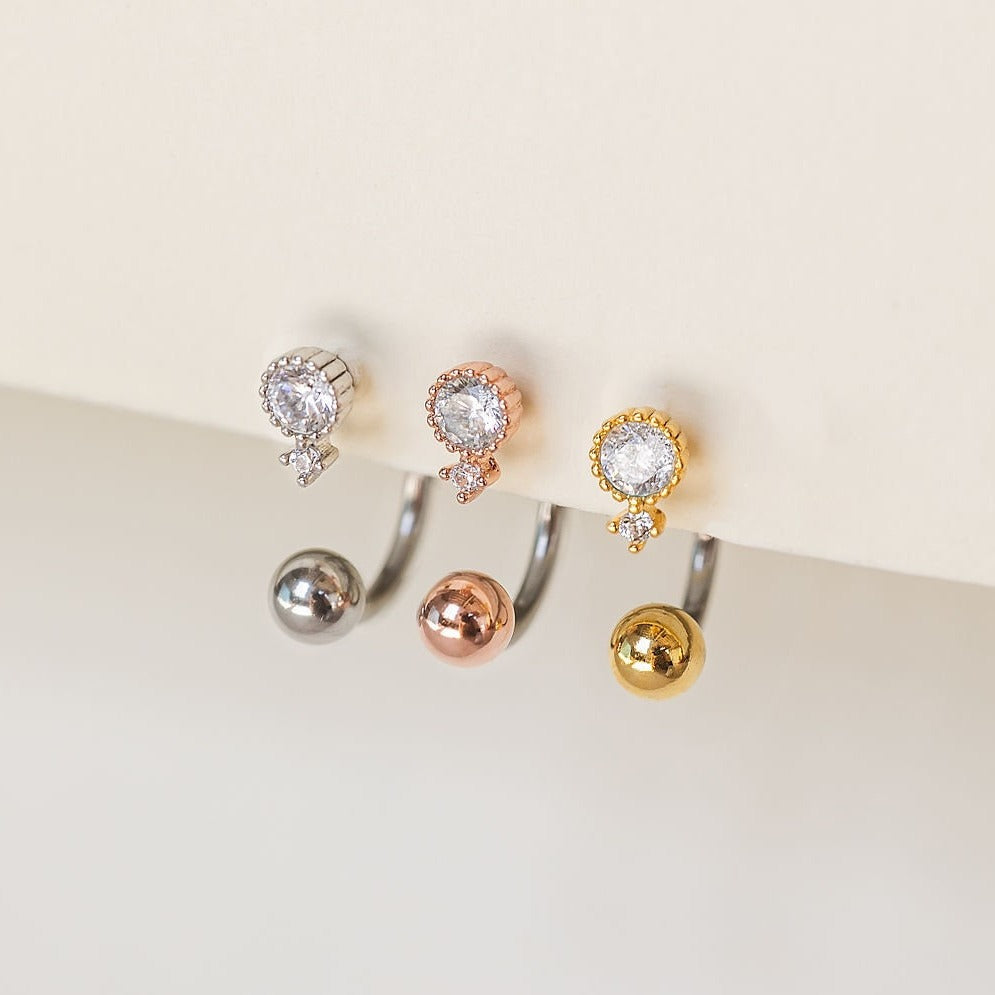The photograph features a set of earrings laid out on a soft white surface, presenting a high level of clarity and detail. At the bottom of the image, there are three curved earrings, each with a distinct metallic hue: a gold earring with a silver backing, a rose gold earring with a silver backing, and a silver earring with a silver backing. Light reflections are noticeable on these metallic surfaces, enhancing their polished appearance. Above these, there are three smaller, non-curved earrings, each adorned with a white gemstone: a gold earring with a white gem, a rose gold earring with a white gem, and a silver earring with a white gem. The soft white background captures the delicate round shadows of the gem-adorned earrings, adding depth to the composition. The overall image is highly crisp and clear, showcasing the intricate details and reflective qualities of the earrings.